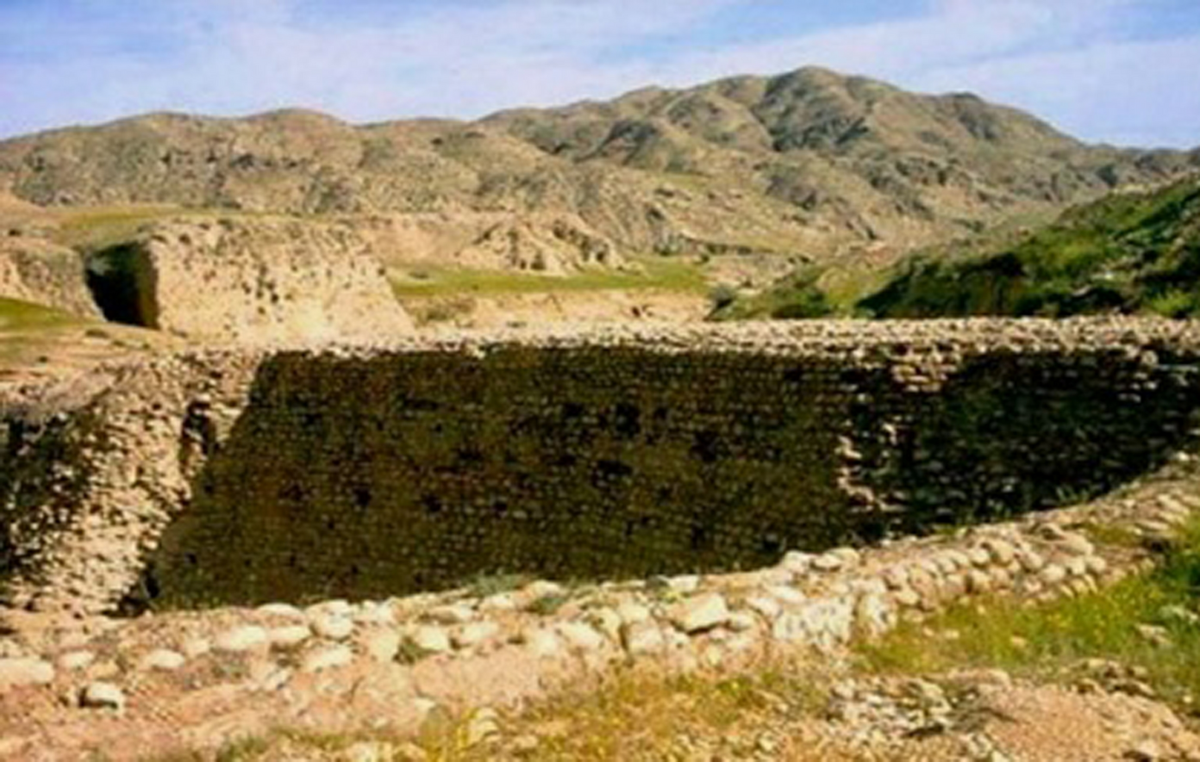The photograph captures a vivid outdoor scene on a sunny day, featuring a hilly, mountainous landscape under a bright blue sky adorned with white clouds. The distant background reveals large mountains about a mile away, while the foreground is dominated by smaller hills. At the center of the image lies a stone-built structure, possibly an archaeological ruin or a retaining wall. The wall spans from the far right to the far left of the image, emerging from the earth with no visible mortar, composed of individual stones roughly the size of small basketballs. This structure, shrouded in shadow on its left side due to the sunlight coming from the top right, contrasts with the surrounding greenery. Brown and green hues dominate the scene, with shades of black accentuating the stones. The patchy grass around the wall and on the hills adds to the natural beauty of this potentially historical ruin, suggesting it may have once served as a reservoir or dam.